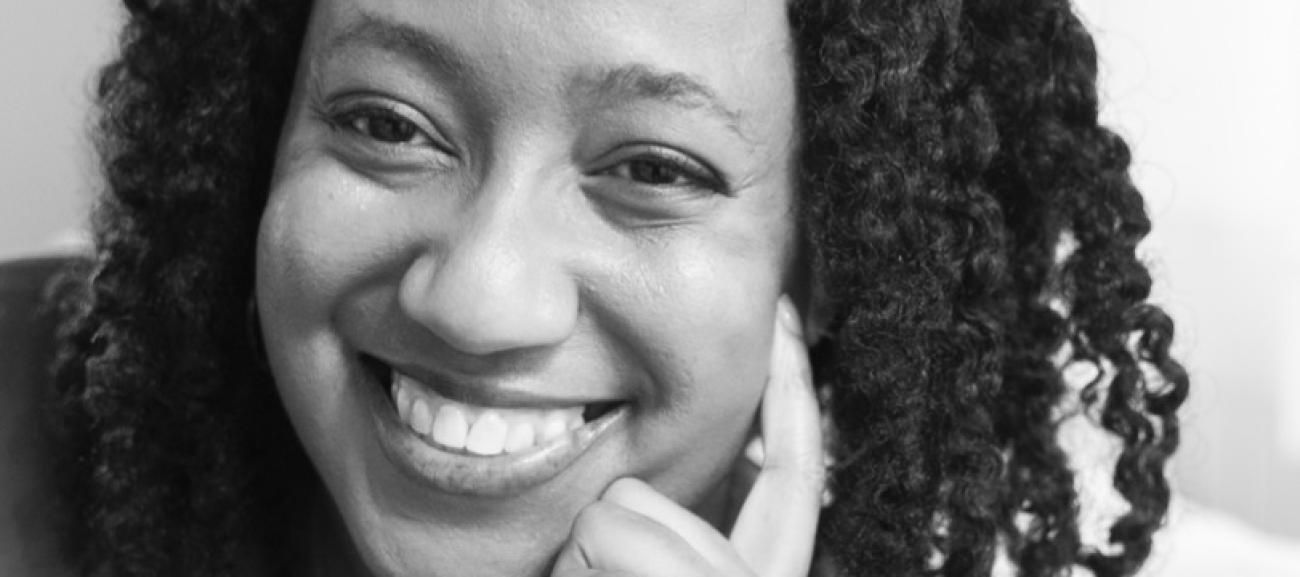This black and white photograph captures a close-up of a smiling woman who exudes a relaxed and familiar aura. Her coarse, curly hair, of a dark hue ranging between brown and black, cascades down to her shoulders. She is slightly off-center, positioned towards the left, with her forehead partly cropped out of the frame. The woman’s bright, wide smile reveals her very white teeth, and her eyes are squinted, adding to the warmth of her expression. Her left hand is delicately positioned against her face; the index finger is pointing up and touching her cheek, while the remaining fingers are gently curled against her chin and jawline. The image showcases her clean yet slightly shaggy eyebrows and hints at her wearing a dark-colored top. Overall, the minimalistic setting, devoid of identifying details, focuses purely on the woman's expressive, serene demeanor.